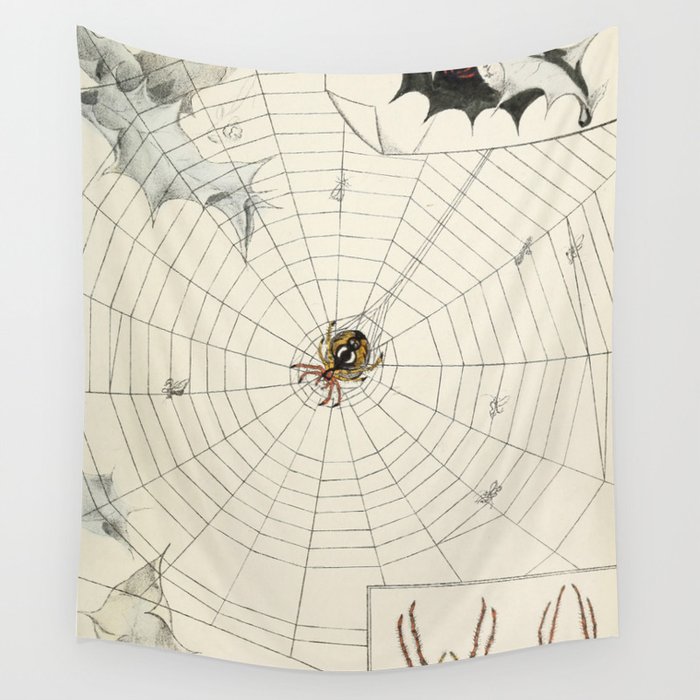The image is a detailed illustration that resembles a tapestry or blanket, featuring a prominent spider web against a grayish-white background with a creamy beige cloth. The web is intricately designed, spreading outward from the center where a large brown spider with an eyeball-like marking on its abdomen is poised, as if waiting for prey. Among the web's strands, various small insects can be seen entangled, adding to the lifelike depiction. The upper edge of the tapestry features striking black and white triangular designs, while the lower right corner shows discernible brown spindly spider legs. Surrounding the web, gray shapes resembling leaves and what appears to be a dog are subtly integrated into the design, enhancing the tapestry's intricate and eerie composition.